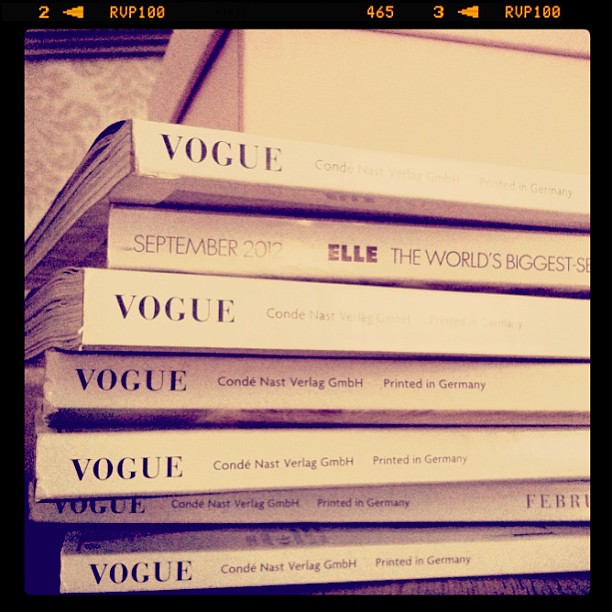The image depicts a square-format, color photograph of a stack of seven magazines viewed from the side, with their titles prominently displayed. At the top of the stack is a white box. Directly beneath it, the second magazine is an issue of Elle from September 2012, labeled as "The World's Biggest." The remaining six magazines are different issues of Vogue, with some marked "Conde Nast," printed in Germany, and one specifically dated February. The photograph has a distinct purplish cast, suggesting heavy editing or an Instagram filter. The entire image is inset in a black border with yellow details, mimicking the look of a 120 square film, noted with "Rup 100," the numbers "2" and "3," and directional arrows. The top left corner features a tapestry border against the background, and the overall style is photographic realism.